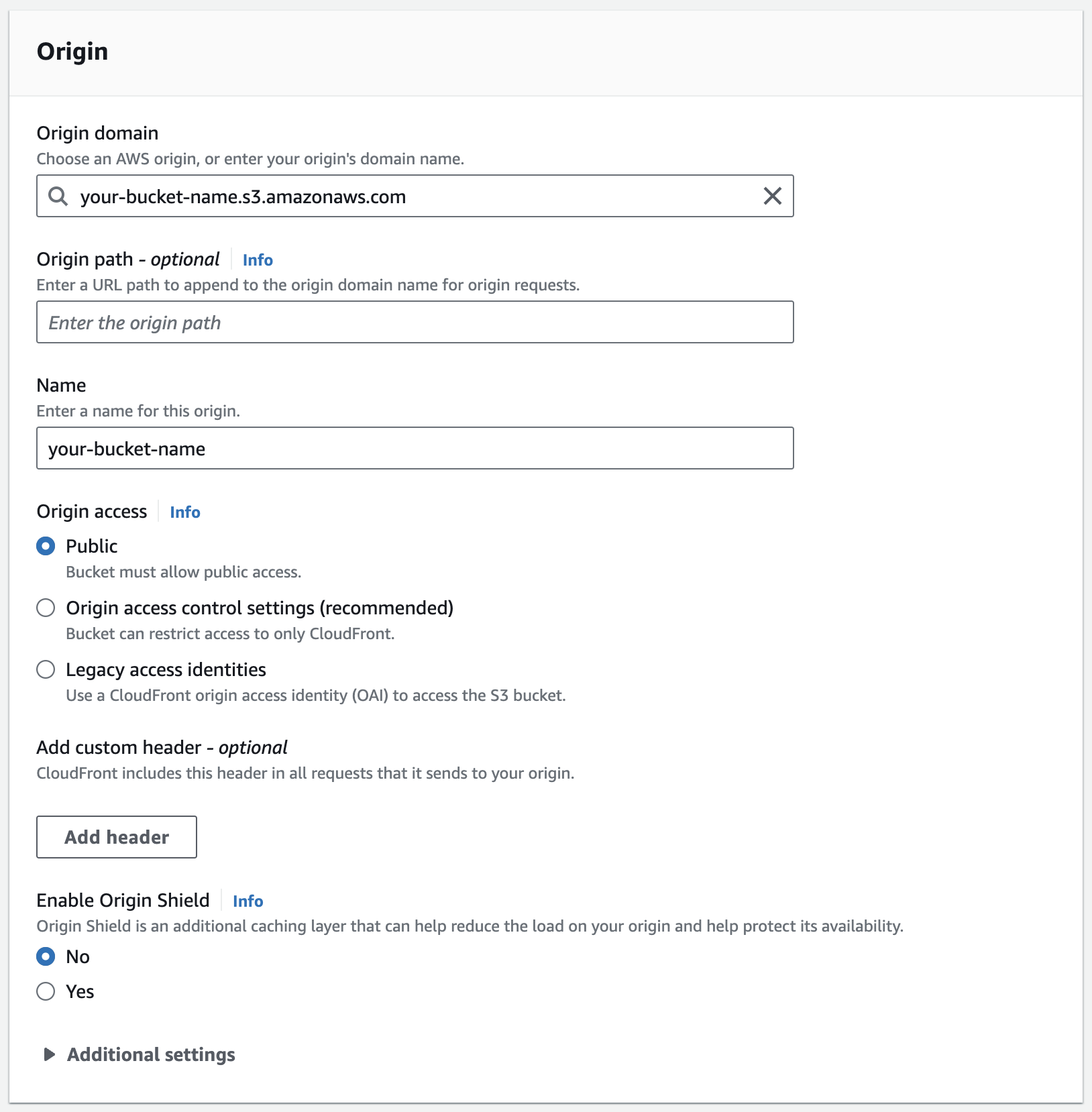The image displays a web page with a predominantly white background, accompanied by black and blue text. At the top, the word "Origin" is prominently displayed in bold black font. Below, the user is prompted to choose an AWS origin or enter their origin's domain name, with the example "your-bucket-name-s3.amazonaws.com" shown in the search bar beside a magnifying glass icon.

Further down, there is a section for "Origin Path" which is optional, highlighted by a blue informational hyperlink. This section allows users to append a URL path to the origin domain name for origin requests, though the field is currently blank.

In the "Name" section, the user is directed to enter a name for the origin, with "your-bucket-name" already filled in within a rectangular input box. Next to this is another blue hyperlink labeled "Origin access info."

Beneath this, there's a "Public" option featuring a circular blue button, indicating that the bucket must match public access settings. Additionally, there are two unchecked circular options labeled "Origin access control settings (recommended)" and "Legacy access identifiers."

Towards the bottom, there's an "Add Custom Header" optional section, followed by an "Add Header" button, displayed as a rectangular button. Each element appears thoughtfully structured to guide the user through configuring their AWS origin settings.